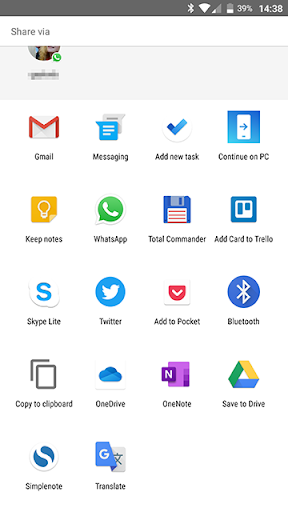A screenshot captured at 14:38 displays the device's battery at 39%. The screen shows a "Share via" menu featuring a variety of app options for sharing, including Gmail, Messaging, Add New Task, Continue on PC, Keynotes, Keep Notes, WhatsApp, Total Commander, Add Card to Task, Add Card to Trello, Skype, Skype Lite, Twitter, Add to Pocket, Bluetooth, Copy to Clipboard, OneDrive, OneNote, Save to Drive, Simple Note, and Translate. The background of the interface is white.